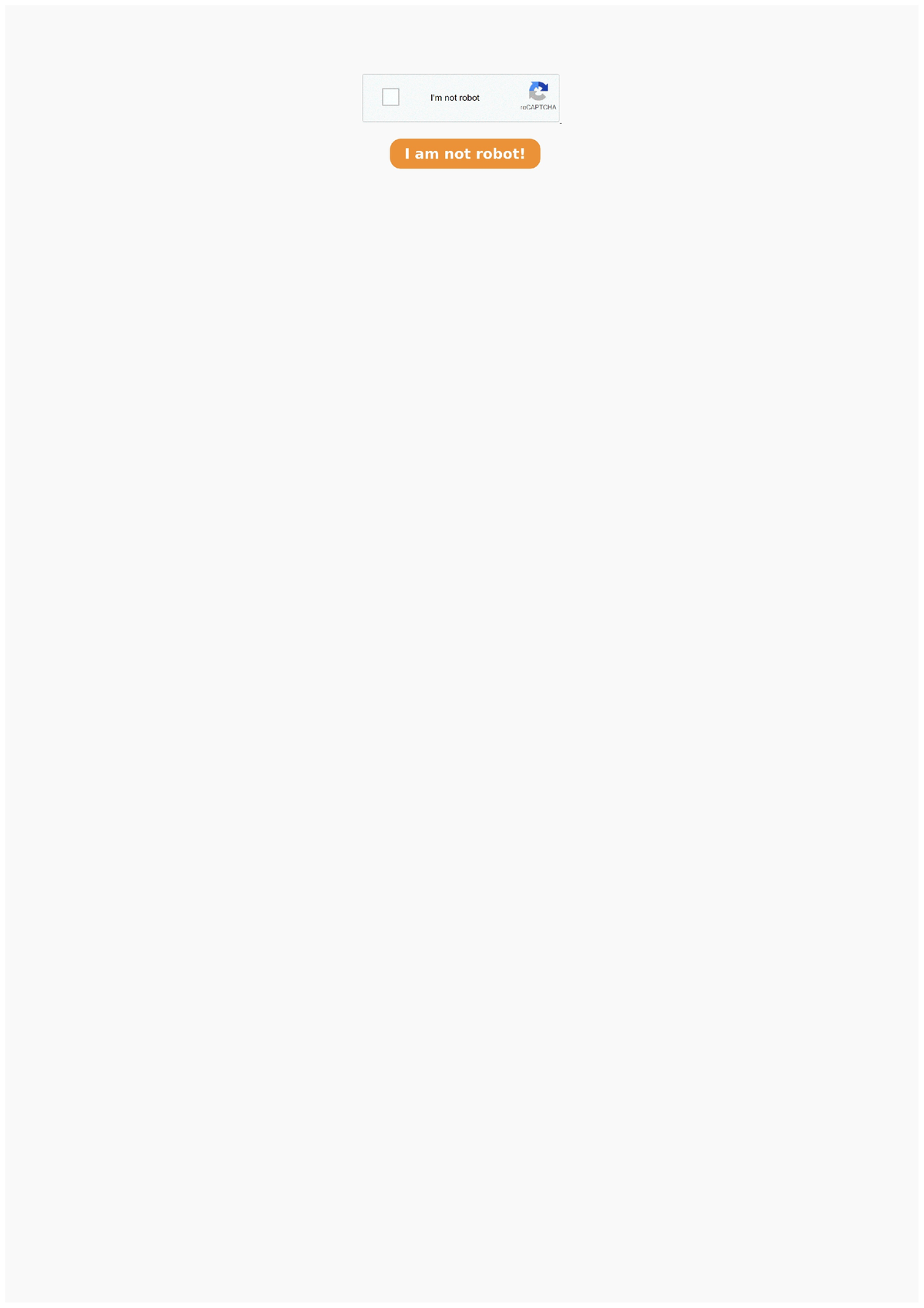This image is a screen capture showcasing a very large, light tan-colored web page. At the top section of the page, there's a login area featuring a CAPTCHA verification process. This section includes a gray box with a white square, inside of which there's black text that is currently not marked. Adjacent to this text is a blue and gray CAPTCHA arrow icon, followed by some additional smaller gray text underneath. The entire CAPTCHA area is enclosed by a thin gray border.

Moving towards the bottom of the image, there's a prominent orange button with white font that reads "I am not a robot." The screen capture is taken from a zoomed-out perspective, making the details inside the CAPTCHA box difficult to discern. The screenshot is clear and not pixelated, but the distant zoom level makes finer text unreadable. The page is devoid of any other images, text, animals, or human elements, leaving the CAPTCHA verification area as the sole focus of the image.